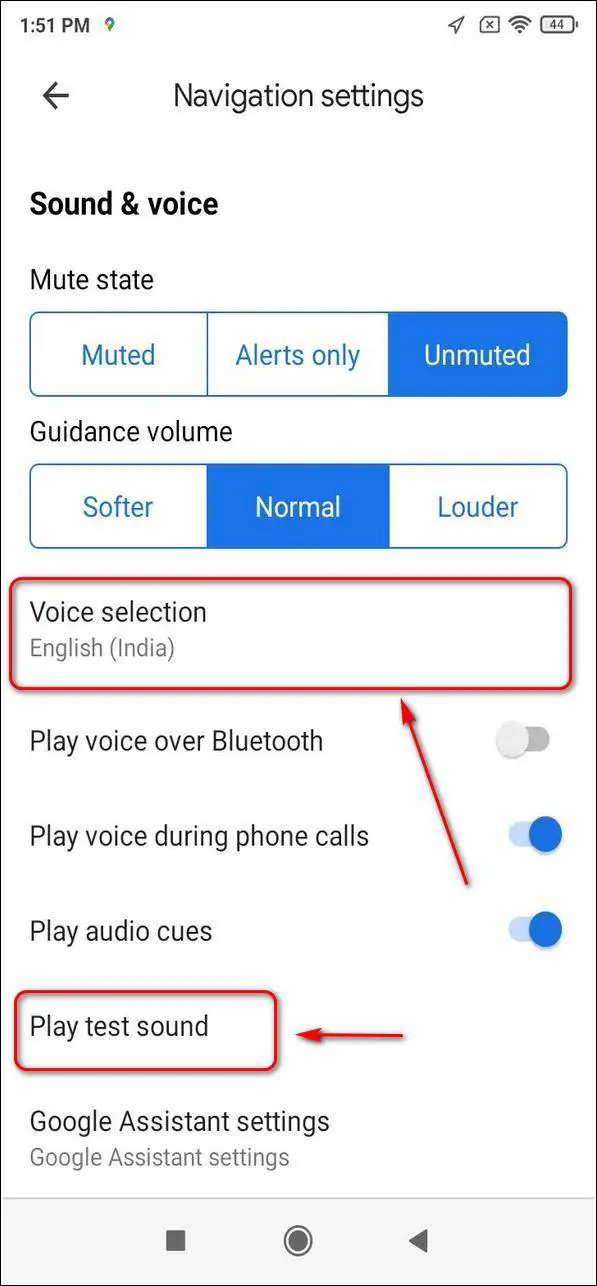This detailed screenshot captures a smartphone interface, specifically from a navigation settings menu, indicating it's currently 1:51 PM with the battery charging, as shown by the lightning bolt icon at the top right. The title "Navigation Settings" is prominently displayed at the top. The left side starts with "Sound and Voice," under which the "Mute State" section lists three options: "Muted," "Alerts Only," and the currently selected "Unmuted," highlighted in blue. 

Following this, there's the "Guidance Volume" category with choices for "Softer," "Normal," and "Louder," where "Normal" is selected. The "Voice Selection" section specifies "English (India)" highlighted with a red rectangle and accompanied by a red arrow, suggesting a preference for English navigation instructions spoken with an Indian accent, likely for Google Maps.

Further down, more settings include "Play voice over Bluetooth" (turned off), "Play voice during phone calls" (turned on), and "Play audio cues" (turned on). The "Play test sound" option is also boxed in a red rectangle with a red arrow pointing at it, indicating possible emphasis. The final setting shown is "Google Assistant Settings," but no further details are provided on this option.